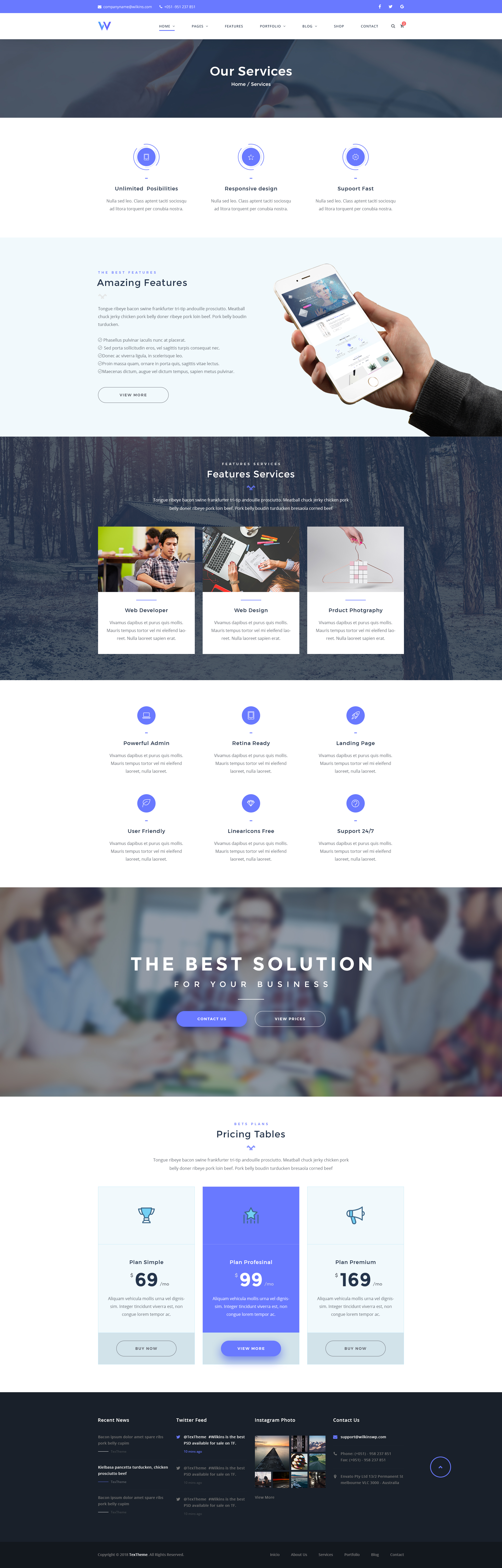This screenshot captures a comprehensive view of an unknown web page designed for a business or service provider. The top navigation bar displays a variety of menu options: "Home," "Pages," "Features," "Portfolio," "Blog," "Shop," "Contact," and "Our Services." Below this, there is a breadcrumb trail reading "Home / Services." The main headline is "Unlimited Possibilities," followed by subheadings such as "Responsive Design," "SupportFast," "The Best Features," and "Amazing Features," with an accompanying "View More" link.

The central visual feature is a photograph of a person’s hand holding a smartphone. Directly below this, different services are outlined:

1. **Features and Services Section:**
   - **Web Developer:** Illustrated with an image of a young man looking at a laptop.
   - **Web Design:** Represented by a photograph of a woman working on a laptop.
   - **Product Photography:** Depicted with an image of a person holding the top part of a wire coat hanger.

2. **Additional Features Highlighted:**
   - **Powerful Admin**
   - **Retina Ready**
   - **Landing Page**
   - **User Friendly**
   - **Linear Icons Free**
   - **Support 24/7**

A promotional statement follows, declaring "The Best Solution for Your Business," accompanied by call-to-action buttons "Contact Us" and "View Prices."

3. **Pricing Tables List:**
   - **Plan Simple:** Priced at $69 per month
   - **Plan Professional:** Priced at $99 per month
   - **Plan Premium:** Priced at $169 per month

Finally, the bottom portion of the image contains some unreadable writing and is largely filled with Latin placeholder text, indicating areas for further content development.